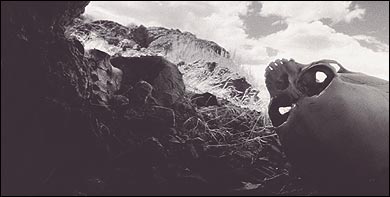The black-and-white image, presented in a rectangular horizontal frame, depicts an eerie and stark landscape. It appears to be a photograph, possibly computer-generated, capturing the inside of a cave. The foreground is dominated by a human skull lying on its side, missing its lower jaw, with the sky visible through its eye sockets. The terrain within the cave is irregular and rocky, darkening progressively towards the deeper parts of the cave. Outside the cave’s mouth, the landscape transitions into a desolate, mountainous horizon under a patchy clouded sky. The rugged mountains in the distance delineate a jagged horizon, suggesting a high-altitude, barren desert setting. There is no visible vegetation, reinforcing the stark, lifeless atmosphere of the scene.